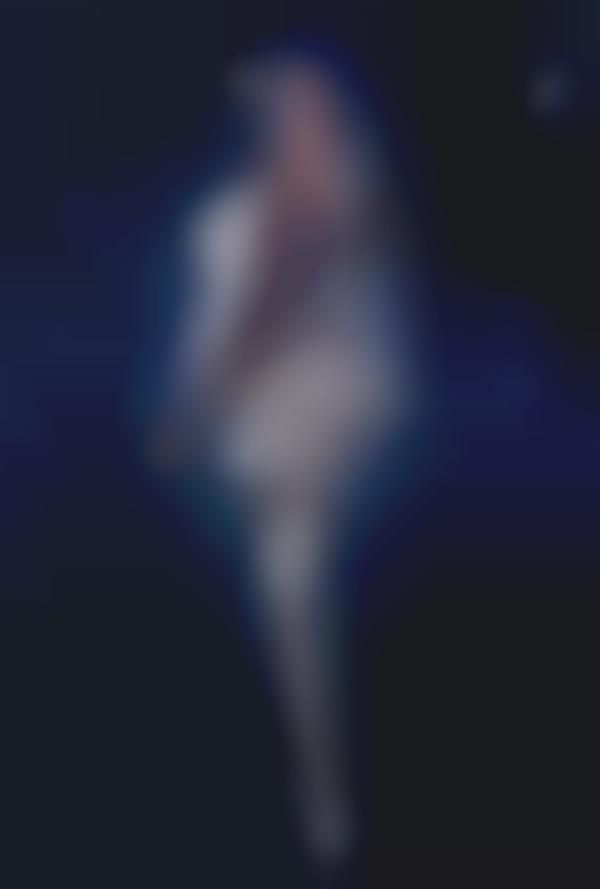This photograph captures a futuristic-themed Barbie doll set against a dark blue, blurred background speckled with light pink and peach-like reflections, giving it a starry, ethereal effect. The doll stands upright, showcasing her tall white leather thigh-high boots that climb past her knees. Above, she dons a shimmering silver skirt adorned with white rectangular patterns, paired with a torso outfit that is white with intricate blue accents. Her attire includes a sheer white jacket with puffy sleeves, complemented by silver pauldrons on her shoulders. The sleeves feature a dual-colored theme, being white on the underside and blue on the outer part. In her right hand, she clutches a golden device and wears two brass rings around her wrist. The doll's visage is striking with glossy, long blue hair styled with a top tie that cascades elegantly down her sides. A blue square is painted over her right eye, accentuating her pink lips and highlighting the overall futuristic, robot-like aesthetic of her attire.